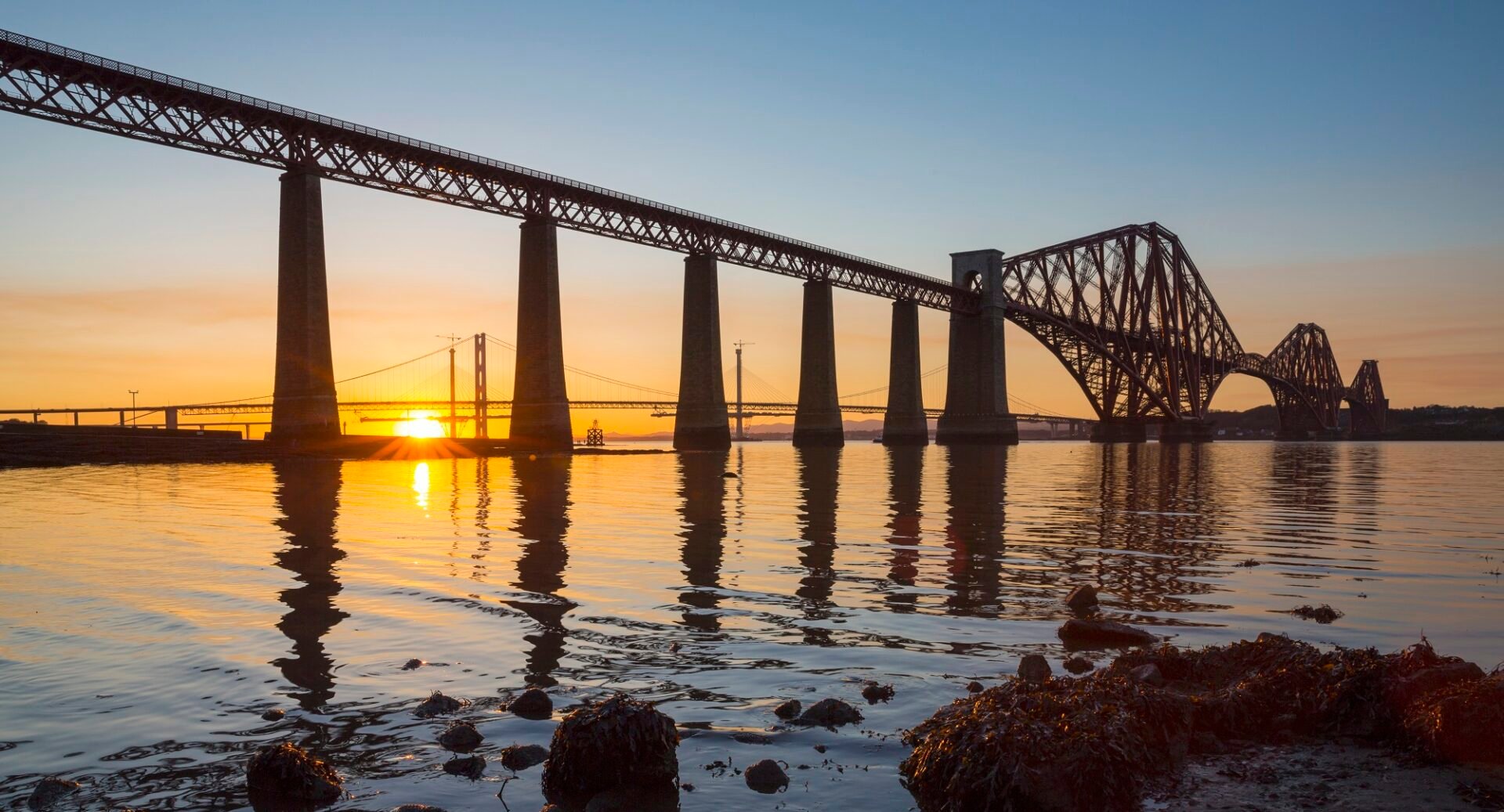This image depicts a vast bridge stretching over a body of calm, reflective water, possibly a river or ocean. The bridge, characterized by its grid-style metal frame and long columns, dominates the scene. It's sunset, with the sky transitioning from blue to orange, and the sun can be seen near the middle left, casting a golden glow and reflecting beautifully in the water. In the distance, another bridge spans the horizon. Close to the shore on the bottom right, clusters of seaweed and rocks are visible, adding to the serene yet intricate details of the scene. The overall composition showcases the bridge's expansive reach and the tranquil beauty of the sunset-lit landscape.